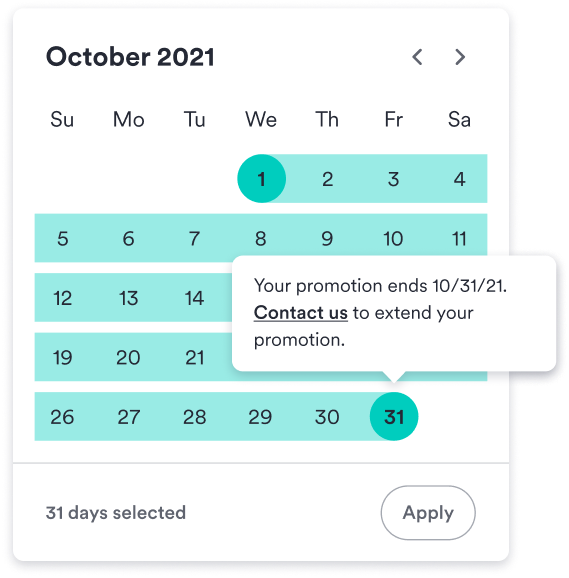This image features a detailed screenshot of a digital calendar interface. The calendar is primarily white with a prominent arrow on the right, providing options to navigate to the previous or next months. Below the navigation arrows, the days of the week are abbreviated as SU for Sunday, MO for Monday, TU for Tuesday, WE for Wednesday, TH for Thursday, FR for Friday, and SA for Saturday.

Aligned under these abbreviations are the dates of the month, starting with Monday the 1st, which is notably highlighted in green. A continuous green bar spans across all dates up to the 31st, which is a Friday. This final date is distinctly highlighted within a green circle. Above the date 31, there's a small text box stating, "Your promotion ends 10/31/21. Contact us to extend your promotion," with "Contact us" underlined and in bold for emphasis.

At the bottom of the calendar, there's an indication that "31 days selected," followed by a white "Apply" button to the right. This concise yet informative image helps users understand the selected date range and provides directions for extending a promotion period.